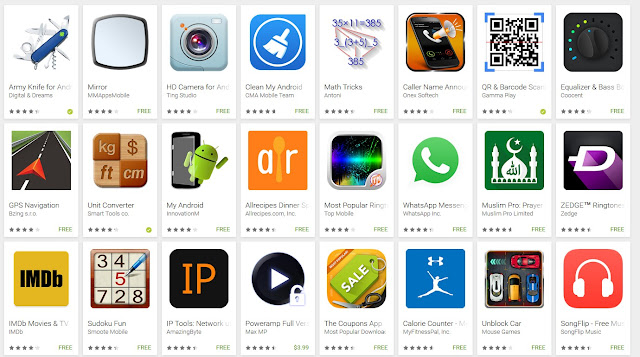This image showcases a diverse array of apps available for download, each rated 4 stars or higher. The selection includes practical tools and entertainment options such as "Army Knife for Digital Dreams," "Mirror," "HD Carries for Android Studio," and "CleanMyAndroid." Utility apps like "Math Tricks," "CallerName," "Equalizer," "BarcodeScan," "GPS Navigation," "Unit Converter," and "MyAndroid" are also featured. Additionally, there are specialized apps such as "AllScripts to Driver," "MostPopularSomething," "WhatsApp Messaging," "Muslim Pro Prayer," "Zedge" for ringtones, and "IMDB Movies." For leisure, there are "Sudoku Fun" and "SongFlip Free Music." Technical users might find "IP Tools Network" and "PowerStamp Full Version" (marked with a lock) useful. Other unique offerings include the "DuPont app," "Cologne Daunter," and "Unblock Car." Nearly all the apps appear to be free, with only one or two exceptions.